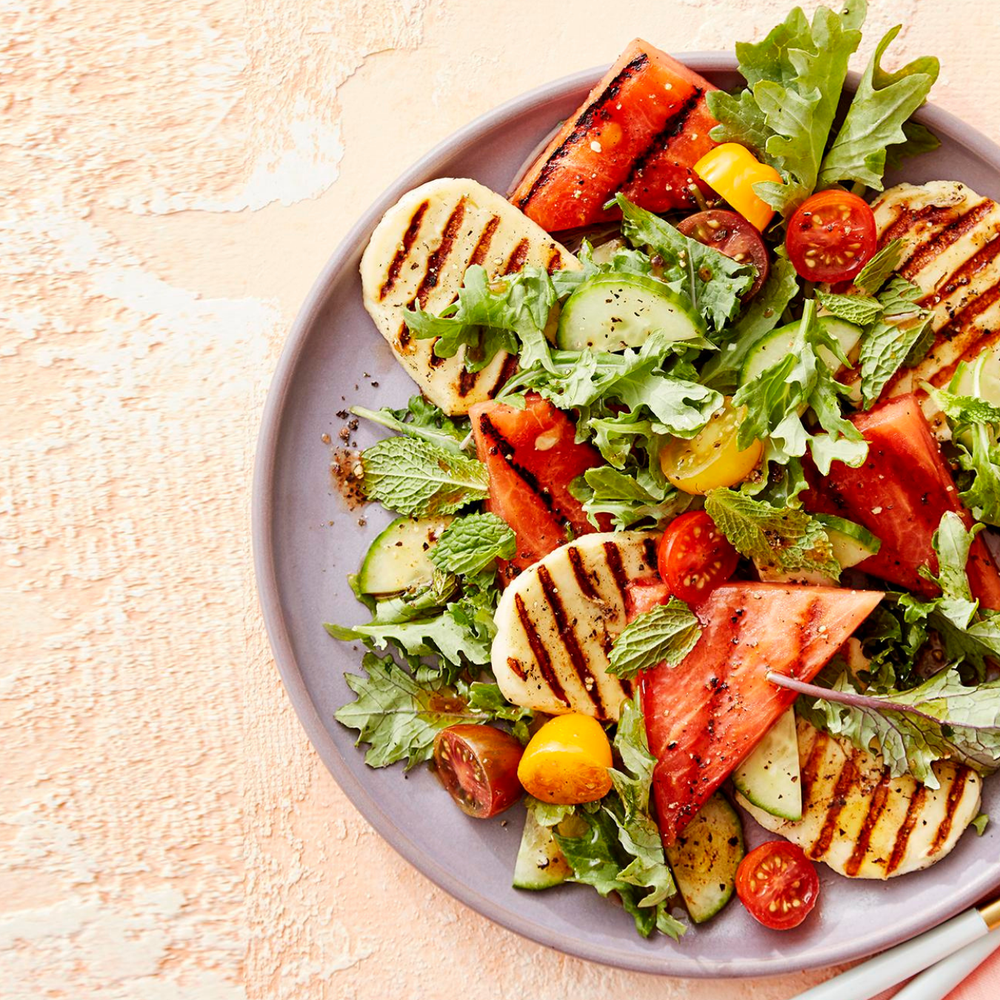The photograph captures a vibrant and richly detailed plate of grilled peach and tomato salad with cannellini beans and a creamy dressing. The salad is artfully presented on a grey, circular plate set on a pale pink tablecloth with a lacy texture. The dish features an array of colors including shades of white, cream, pink, red, green, and yellow. 

The ingredients include arugula, mint, cherry tomatoes (both red and gold), and sliced cucumbers. The tomatoes are halved, while some larger ones are grilled. Grilled items, such as red pepper slices and possibly chicken breasts or bread, are also included, displaying distinct grill marks. The entire plate is seasoned and garnished, creating a visually appealing and appetizing dish.